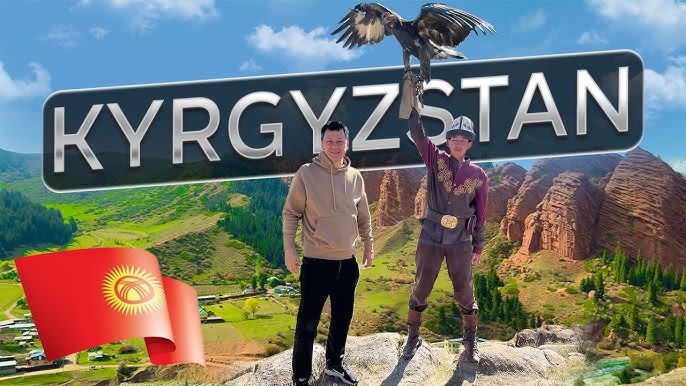This image captures two male travelers standing on a rock against the sweeping natural backdrop of Kyrgyzstan. The photograph is superimposed with a graphic that reads "Kyrgyzstan" in large silver letters on a black background. To the right, there is a scenic view of a red, layered clay mountain range, while the left side features greener hills with patches of forest. The sky above is blue with a few clouds, indicating a clear, sunny day.

The man on the right is dressed in traditional attire, including leather or brown canvas pants, a black outfit that features a large gold belt buckle, and a distinctive hat resembling a silver bell. He holds a large bird of prey, possibly an eagle or a condor, on his right hand, protected by a thick glove. This suggests he might be a falconer. The second individual, to the left, wears a contemporary tan hoodie, dark pants, and black tennis shoes, with short black hair.

Prominently displayed in the foreground is the national flag of Kyrgyzstan, which is red with a yellow sun surrounded by 40 rays and a yellow circle containing three intersecting lines, likely meant to represent the traditional yurt. Together, the individuals and the added elements give the impression that this might be an advertisement for travel or tourism in Kyrgyzstan, highlighting its rich culture and majestic landscapes.